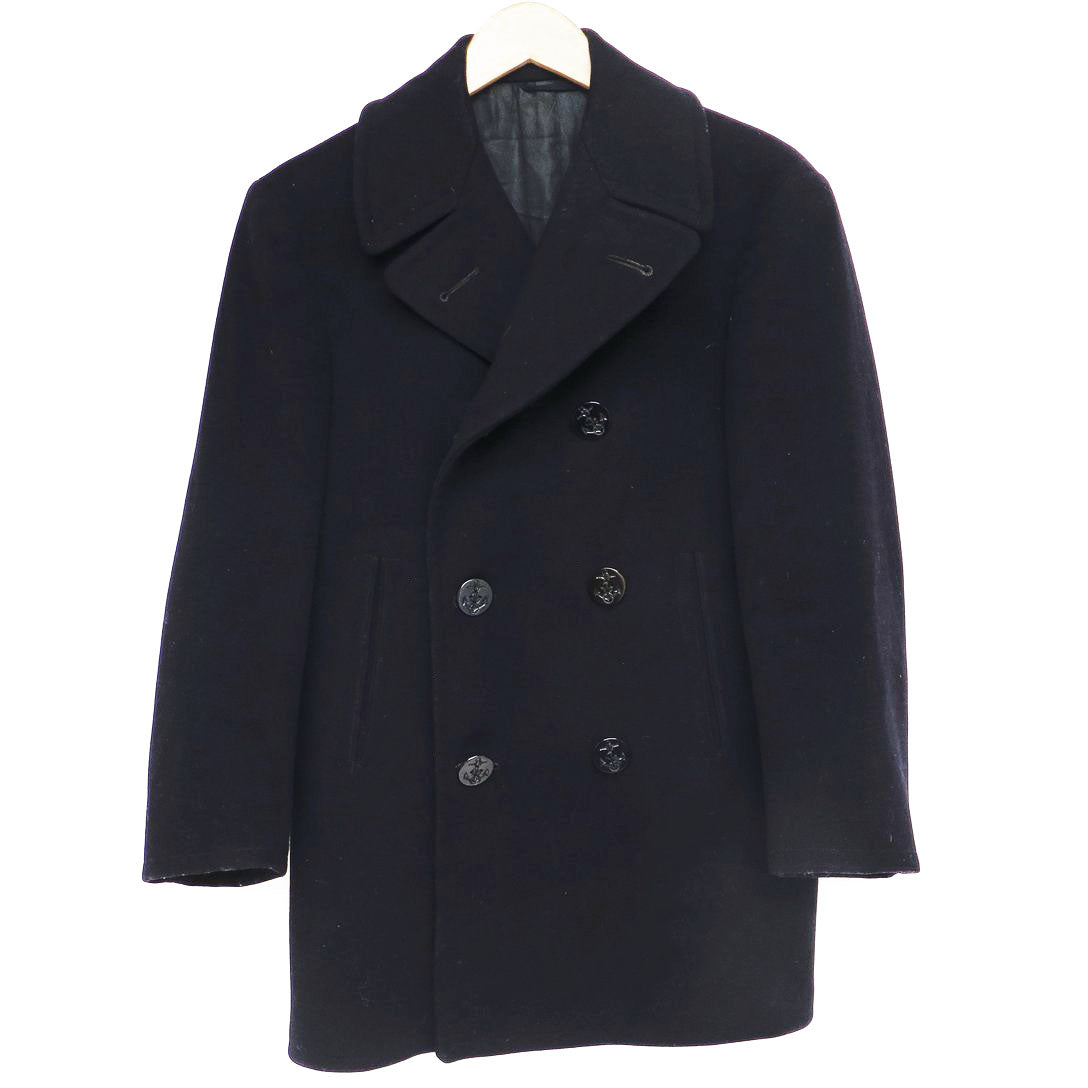The photograph showcases a black, woolen, double-breasted peacoat designed for a small child. This elegant jacket, hanging against a pure white background on a white hanger, features six glossy black buttons arranged in three rows on the front, aligned with a dressy style inner lining. The buttons, each adorned with anchors, complement the peacoat's nautical flair. The jacket's design is further accentuated by its extremely wide lapels, each containing an additional buttonhole. The peacoat boasts two side pockets and long sleeves, suggesting it is suitable for winter. The hem is meticulously tapered towards the left side, providing a tailored appearance, while a peek of the same black lining is visible where the neck is formed by the lapels. A small segment of the inner lining is visible at the back center top of the jacket.